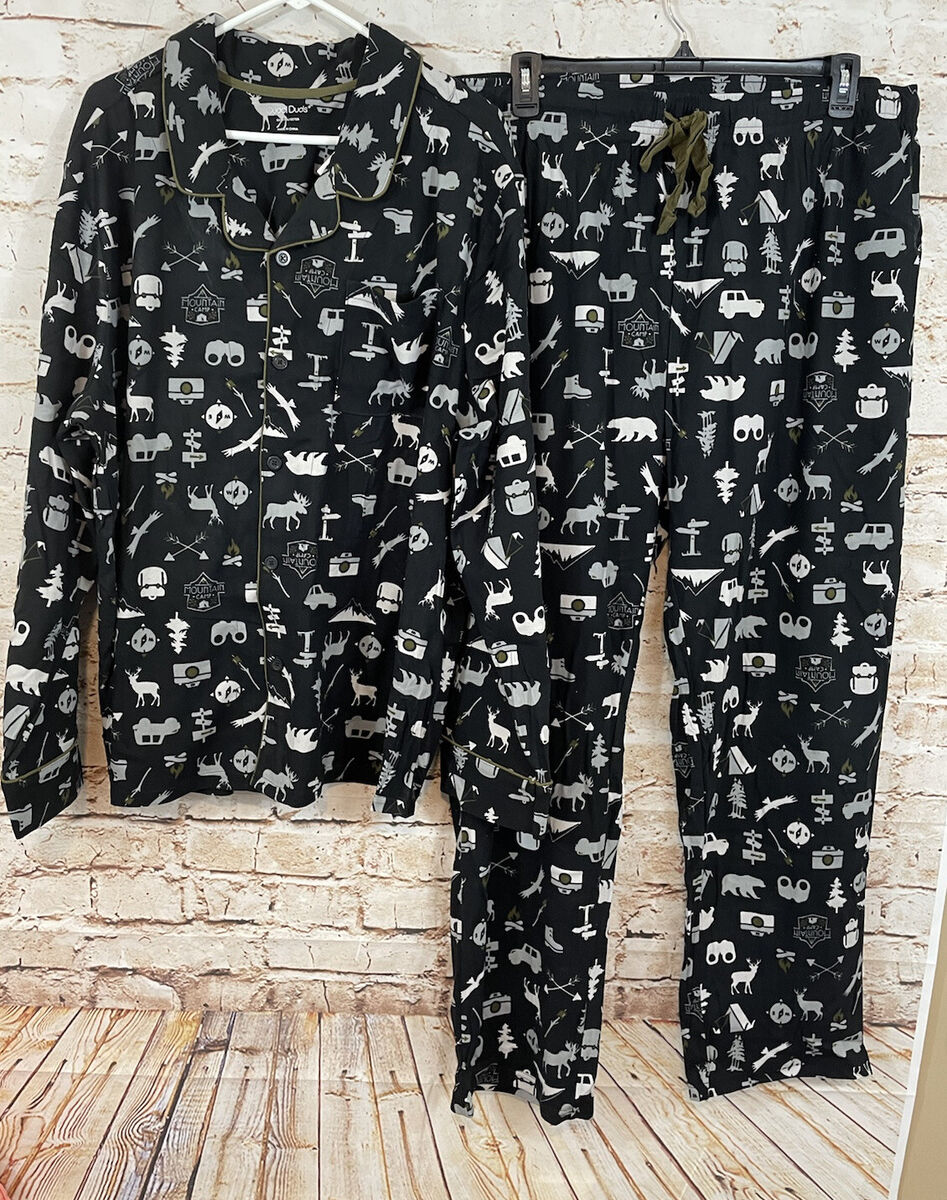The image portrays a rectangular photograph of a pair of unisex pajamas, seemingly taken as a photograph of a photograph. The bottom right corner shows the edge of the original photograph, outlined in white with a beige background. The pajamas are displayed on two separate hangers against a tan-colored brick wall, which is complemented by a similarly hued wood floor. The pajama set consists of a long-sleeved, button-down shirt on a white plastic hanger and drawstring waist pants on a black plastic hanger, both in a solid black fabric adorned with a busy white print. The intricate design features an array of outdoor-themed icons such as polar bears, moose, jeeps, houses, upside-down trees, arrows, binoculars, and compasses. These varied motifs create a lively and detailed pattern across the pajamas, emphasizing their distinctive, outdoorsy aesthetic.